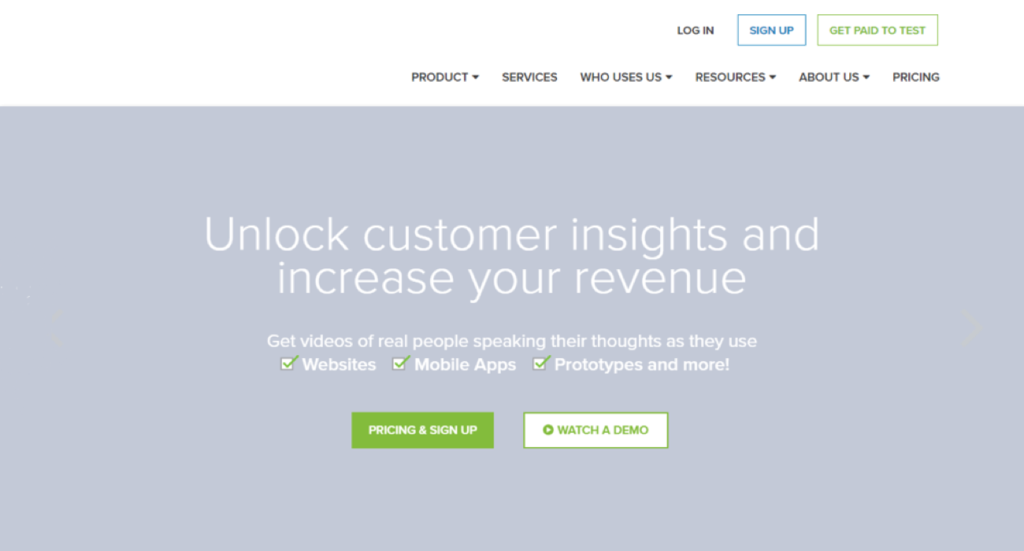**Homepage of a User Testing Platform**

The homepage of the user testing website features a clean and user-friendly design with a light gray background. A prominent white banner stretches across the top of the page, containing a well-organized set of navigational links. Centrally located at the top are the menu items: "Product," "Services," "Who Uses Us," "Resources," "About Us," and "Pricing," each accompanied by a drop-down menu for easy access to subcategories.

To the far right of this navigation bar, there is a "Login" link. Adjacent to it, a blue-outlined rectangle with blue text encourages visitors to "Sign Up." Next to this, a light gray-outlined rectangle features green text inviting users to "Get Paid to Test."

Dominating the main section of the light gray background is an inviting headline in white text: "Unlock Customer Insights and Increase Your Revenue." Beneath this headline, a subheading in smaller white text reads, "Get videos of real people speaking their thoughts as they use websites, mobile apps, prototypes, and more." Three key areas—websites, mobile apps, and prototypes—are highlighted with little white checkboxes and green check marks, emphasizing the platform’s testing capabilities.

Below the text are two side-by-side call-to-action rectangles. The left rectangle is green with white text, stating "Pricing and Sign Up." The right rectangle is white with green text and includes a directional arrow that says "Watch a Demo," guiding users to explore more about the service.

This detailed layout and clean design make the homepage visually appealing and easy to navigate, guiding users smoothly through their journey on the website.